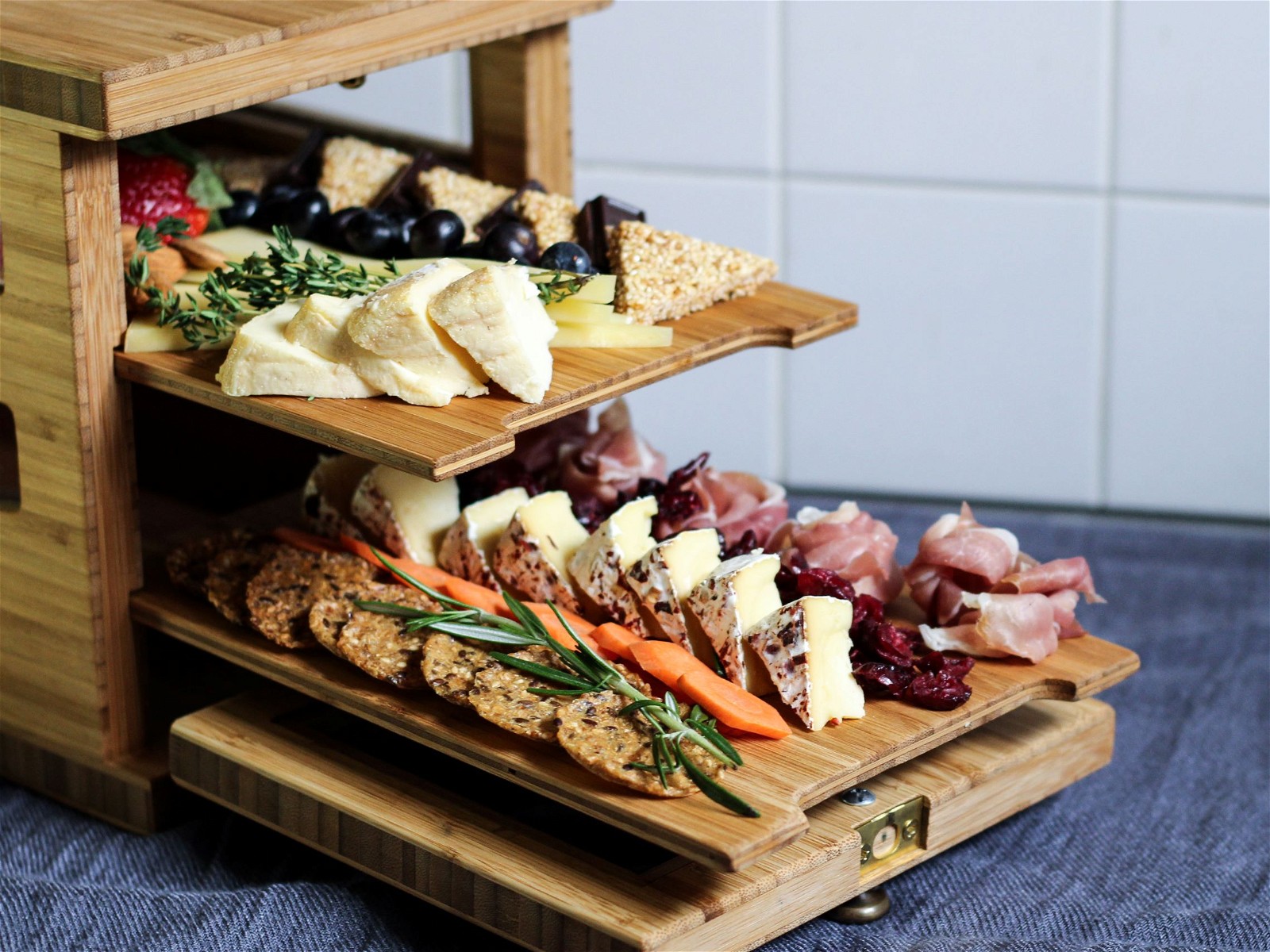The image depicts a professional photograph of a wooden, two-tiered charcuterie board designed to slide out from a picnic basket-like shelf. The boards, placed on a blue tablecloth, are adorned with an assortment of fine cheeses, thinly sliced meats, dried fruits, and fresh produce. The top layer features various cheese slices, including mozzarella and yellow-whitish varieties, alongside strawberries and blueberries. The bottom layer includes an array of unique textured cheeses, thinly sliced meats, crackers with herbs (possibly rosemary), and fresh vegetables such as carrots. Additional items like berries and what seems to be sesame seed-covered crackers are also present. In the background, a large white tile backsplash adds a clean, bright contrast to the richly textured display.